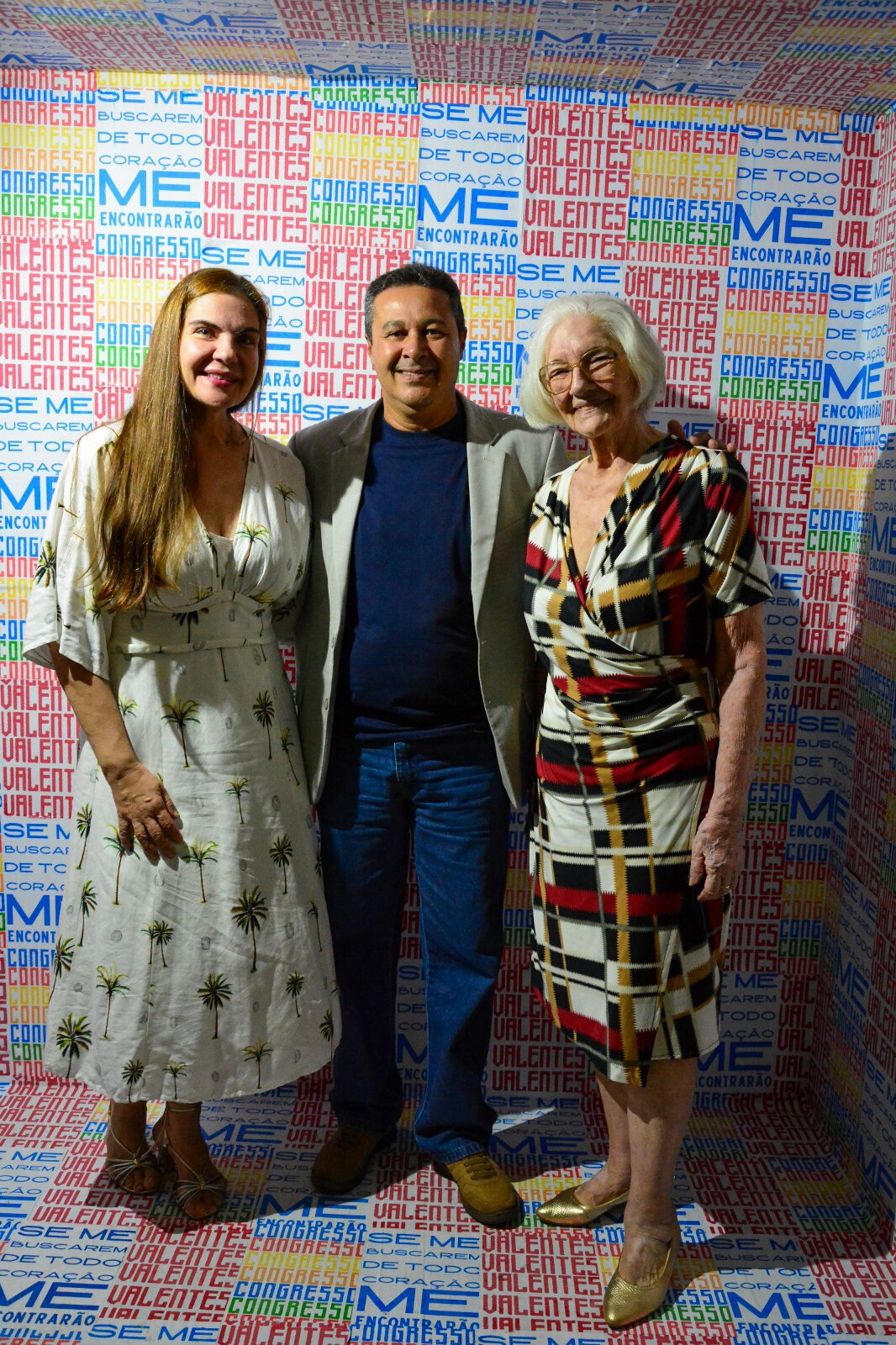The photograph captures three individuals standing together and smiling at the camera, appearing to be at an event, possibly a political or art-related one. The backdrop prominently displays the words "Valentins Congresso" in various colors and sizes, suggesting a vibrant and festive atmosphere. 

On the left is a woman in her late 50s or early 60s with long, light brownish-blonde hair. She is dressed in a white ankle-length dress adorned with small palm trees and is wearing either sandals or heels. Next to her, in the center, is a man who could be Latino. He is dressed in a combination of a white suit jacket over a blue sweater, blue jeans, and brown shoes, giving off a casual yet polished appearance.

On the right is an elderly woman, likely in her 70s or 80s, with white hair and glasses. She is dressed in a colorful dress reminiscent of a Picasso painting, featuring a mix of white, red, and gold, and she completes her ensemble with golden shoes. All three individuals convey a sense of joy and unity, presumably supporting a significant occasion or campaign for Valentins Congresso, as indicated by the repetitive signage in the background.